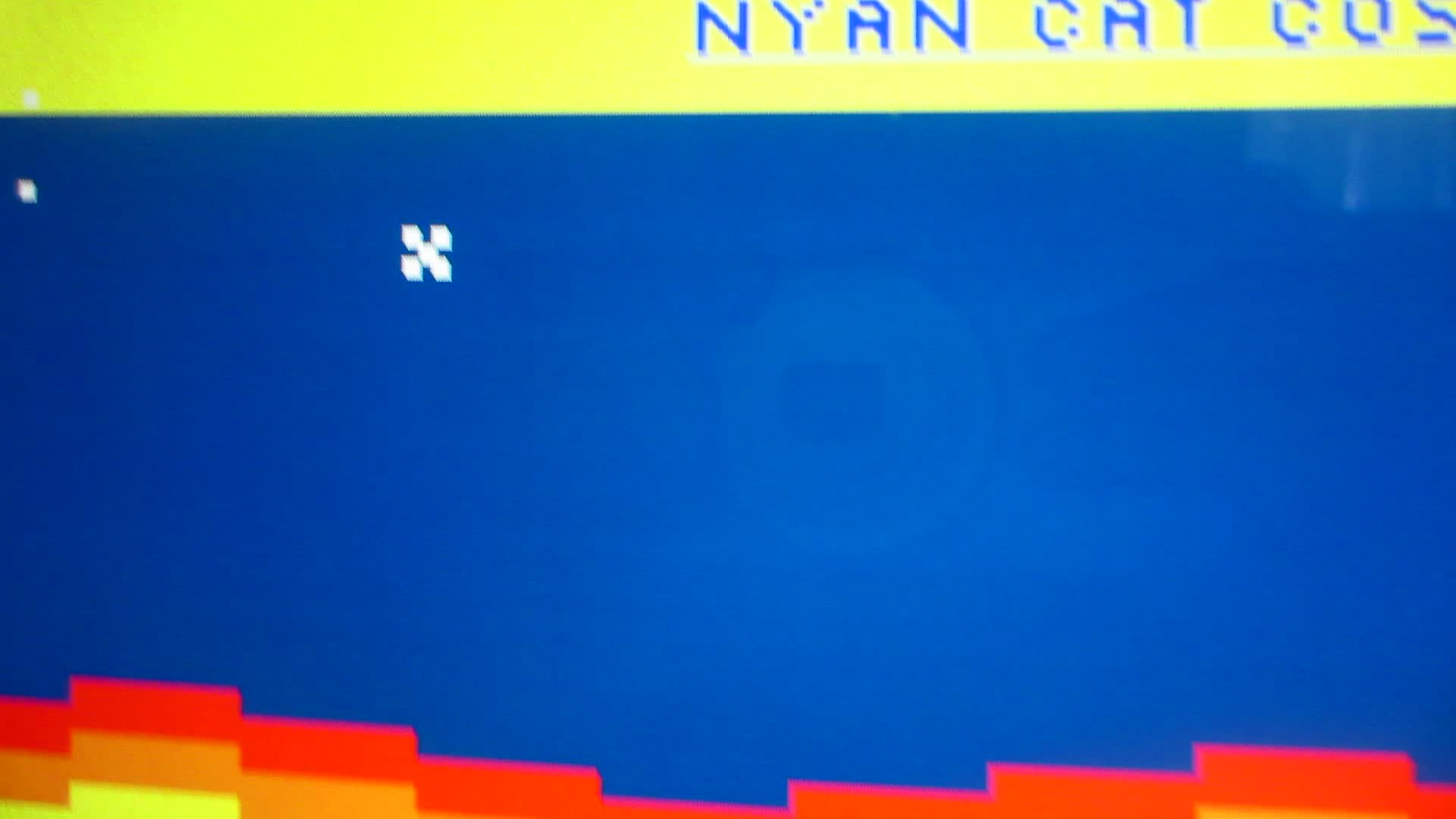This is a detailed screenshot from a video game, portraying a somewhat blurry and simplistic capture of a computer screen. Dominating the image is a dark blue background with slight discoloration towards the center. At the top, there is a yellow banner that reads "Nyan Cat C.O.S.," although the text is cut off and all in bright blue letters, accompanied by a small white underline beneath it. The most prominent feature on the screen is a white X-shaped icon composed of five squares—four positioned at the corners and one in the center, slightly offset due to the pixel density of the game. To the left, a small white dot can also be observed in the corner. On both edges of the blue area are vertically stacked rectangles: on the left, they form a sequence of red, orange, and yellow sections, while on the right only the red and part of the orange sections are visible, all creating a pixelated, colorful border reminiscent of the rainbow trail famously associated with the Nyan Cat meme. Additionally, there appears to be a faint reflection within the blue region, adding to the screen's textured appearance.